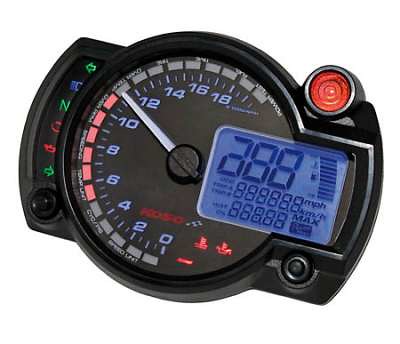The image depicts a sleek, black, rectangular device resembling a speedometer. The device has smoothly rounded edges on the left and right sides, with a circular section in the middle featuring numerical markings. The numbers, ranging from 0 to 18, are arranged in a semicircular pattern starting from the bottom middle of the circle. The numbers 0 through 4 are accompanied by gray rectangular segments below, while numbers 6 through 11 are highlighted with red rectangular segments beneath them, indicating a caution or redline zone. Numbers 11 through 18 have gray rectangles above them, marking the higher end of the scale.

On the right side of the circular dial, within the rectangular frame, there is a blue screen displaying numbers in dark blue text, which appear somewhat fragmented, possibly indicating a reading of "288." The blue screen also shows various ascending ticks, resembling a gas meter, with a repetitive sequence of the digit 8 lined up in multiple rows: six rows on the top and five at the bottom.

Adjacent to this screen, the abbreviations "MPH," "KM/H," and "max" are displayed, signifying the potential units of measurement for the device. Above this section, a red indicator light is visible, suggesting an alert or warning signal.

On the left side of the device, near the edge of the rectangle, there are several illuminated symbols including: a green check engine light, a blue high beam indicator, a green “N” symbol, a red circular warning light, a red oil check indicator, and a green arrow pointing to the right. These symbols likely indicate various statuses or alerts related to the device's function or the vehicle's performance.